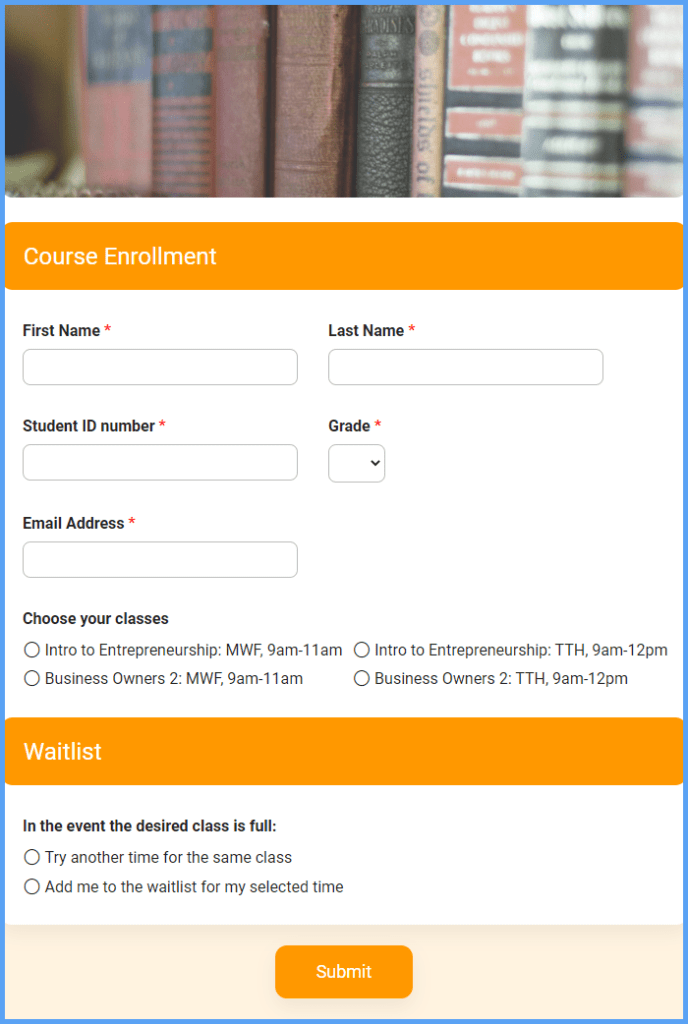The image depicts an online course enrollment form with a structured layout. The form is encased in a blue rectangular border. At the top of the form, there's a bookshelf partially in view, filled with indistinguishable books. Upon closer inspection, one of the book titles appears to be "SHIELD" in an old-style font, but the other titles remain blurry and unreadable. 

Below the blue border, a white section emerges, accompanied by an orange border. On the left side of this section, the words "Course Enrollment" are clearly printed in white, each word capitalized. The background throughout this enrollment form is predominantly white, with various sections needing input from the user.

The input sections are clearly segregated. The form requires a "First Name," "Last Name," "Student ID Number," and "Grade," each marked with a red asterisk, indicating required fields. Additional options appear once scrolling down, including a dropdown black arrow for selecting grades.

The form continues, requiring an "Email Address," again marked with a red asterisk. Following this, the user is prompted to "Choose Your Classes." There are four radio button options available, detailed as follows:
1. Intro to Entrepreneurship, MWF (Monday, Wednesday, Friday) from 9 a.m. to 11 a.m.
2. Business Owners 2, MWF (Monday, Wednesday, Friday) from 9 a.m. to 11 a.m.
3. Intro to Entrepreneurship, TTH (Tuesday, Thursday) from 9 a.m. to 12 p.m.
4. Business Owners 2, TTH (Tuesday, Thursday) from 9 a.m. to 12 p.m.

Following the class selection section, there's another orange border, and within it, the word "Waitlist" is highlighted in white. Beneath this, the instructions in black state that if a desired class is full, the user has two options: try another time for the same class or add to the waitlist for the selected class.

At the bottom of the form, an orange rectangular button stands out with the word "Submit" prominently displayed in white. The overall layout is organized and user-friendly, guiding the user through the necessary steps to enroll in their desired courses.